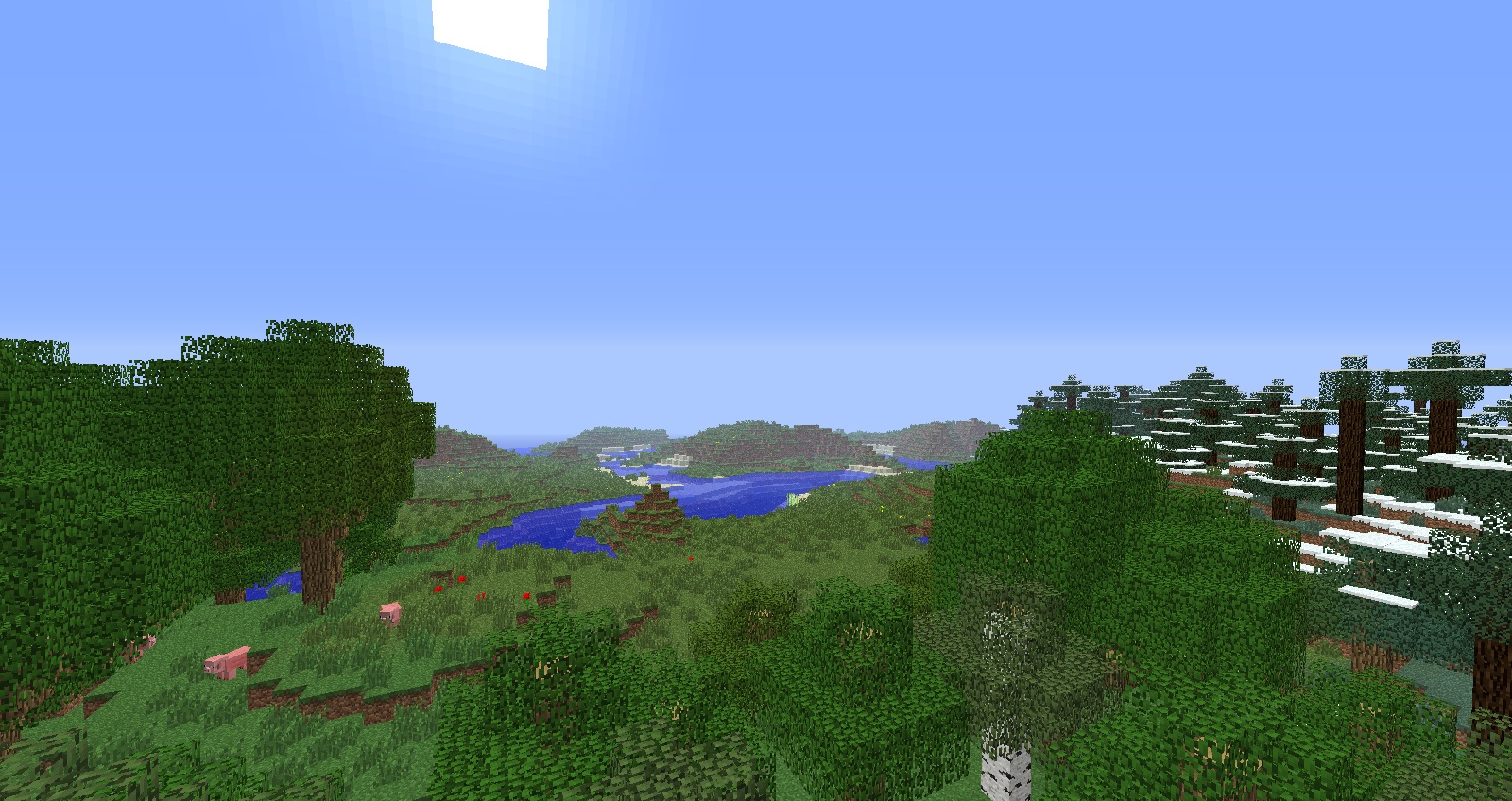The image depicts a pixelated, computer-generated scene resembling an old-school video game landscape. The overall aesthetic is blurry, showcasing individual pixels and a lack of crisp definition, reminiscent of early CGA graphics. Dominating the scene is a blue sky with a conspicuous white chunk, possibly representing a sun with an unusual, diamond-like shape partially off the screen. The terrain is characterized by subtle hills and various shades of green, indicating a valley floor with low scrub brush and mature trees with brown trunks to the left. These trees are prominent despite the pixelation. In the background, there are bodies of water, including a cobalt blue lake fed by a river, located towards the left.

The landscape also features small pinkish figures, likely pigs or possibly cows, scattered across the greenery. Towards the right side, the scene includes a maze-like garden leading to structures made of tree trunks with intricate tops, some of which are dusted with snow. Additional elements include white and black buildings or structures and stones dotted around the grassy fields. Additionally, a brown step-like pyramid outcrop is visible near the water. Red flowers add spots of color on the ground, enhancing the detailed, though pixelated, outdoor environment.